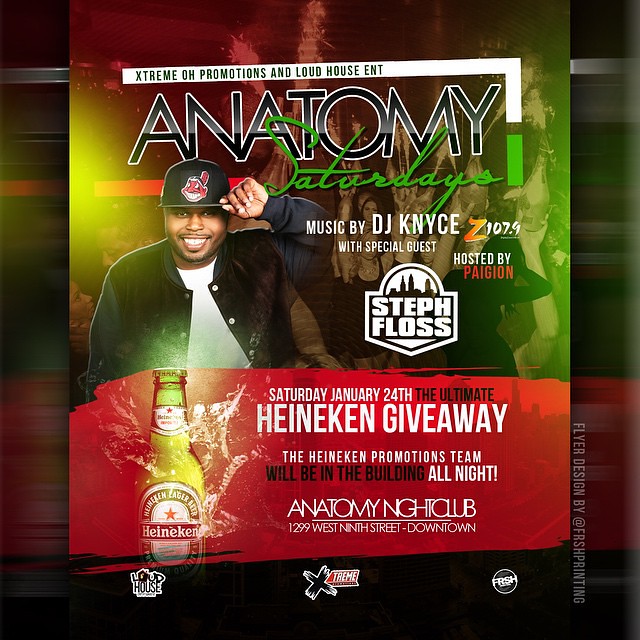The promotional poster features a predominantly black background, which is faintly mirrored by the main image in the forefront. Central to the image is the text "Extreme OH Promotions and Loud House ENT" at the top. The poster prominently displays the word "Anatomy" in bold black font with white borders, and "Saturdays" is written in green cursive below it. On the left side, there is a picture of a man wearing a Cleveland Indians hat, tipping it with his left hand. He is dressed in a black coat with blue sleeves over a white t-shirt. To the right of him, the poster details "Music by DJ Nice (KNYCE)" from Z107.9, with special guest Steph Floss, and it's hosted by Pyjeon (stylized as PA IG Ion) in red.

At the bottom left corner, there's an image of a Heineken beer bottle with water splashing around it. A red strip of background lies beneath, featuring the text "Saturday, January 24th, the ultimate Heineken giveaway. The Heineken Promotions team will be in the building all night at Anatomy Nightclub, 1299 West 9th Street, downtown." Multiple logos, including Loud House, Extreme, and Fresh, are scattered across the bottom of the poster. Additionally, the right-hand side acknowledges, "flyer designed by @Fresh Printing."

This highly detailed summary combines elements from both captions to offer a comprehensive description of the poster.